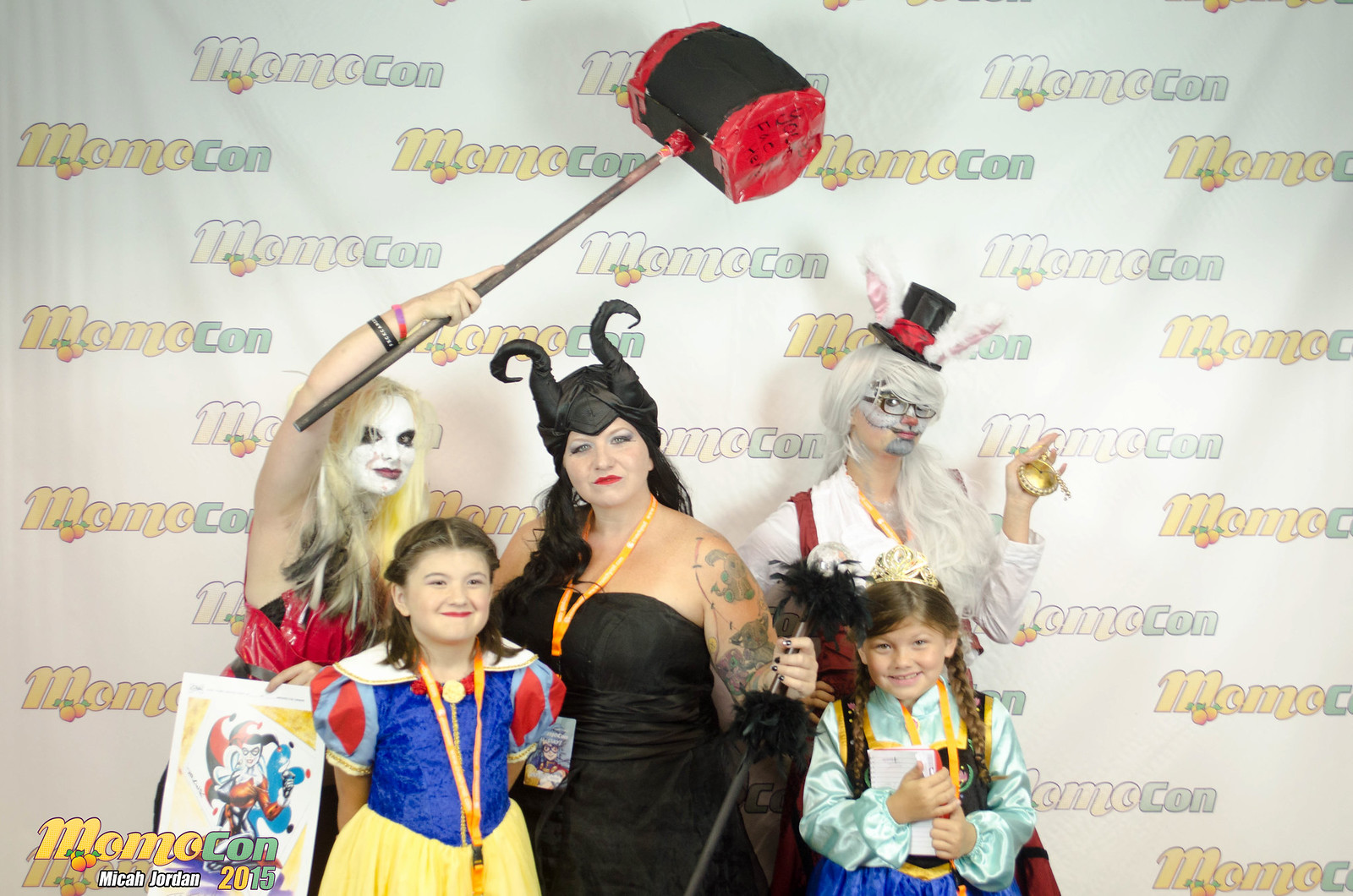In this vibrant and lively photograph taken at MomoCon, a comic book and anime convention indicated by the repeated press banner with a peach-themed logo, we see a diverse group of cosplayers showcasing their elaborate costumes. On the far right stands a young woman cosplaying as Harley Quinn from the Batman series, brandishing a large, black and red circus-style mallet inscribed with "Your Face Here." She is adorned with a blonde wig, striking white face paint, black eye makeup, and red lipstick, embodying the mischievous villainess. To her left, at the front, kneels a little girl dressed in a classic Snow White costume, complete with a ribbon around her neck and braided hair, smiling brightly. Behind Snow White, another layer of detail reveals a woman dressed as Maleficent from Disney's Snow White, distinguishable by her black, horned headpiece and a black strapless dress, her arms accented with tattoos and a ribbon lanyard around her neck. Next in the sequence, a young girl dressed in a blue outfit, possibly resembling Jasmine from Aladdin, adds a touch of royalty with her crown. Finally, to her right, an older woman channels the White Rabbit from Alice in Wonderland, sporting a gray wig with a small top hat adorned with bunny ears, her face painted to complete the rabbit's look, and accessorized with a timepiece. Together, these cosplayers create a tableau of beloved characters, celebrating their fandom with creativity and flair.